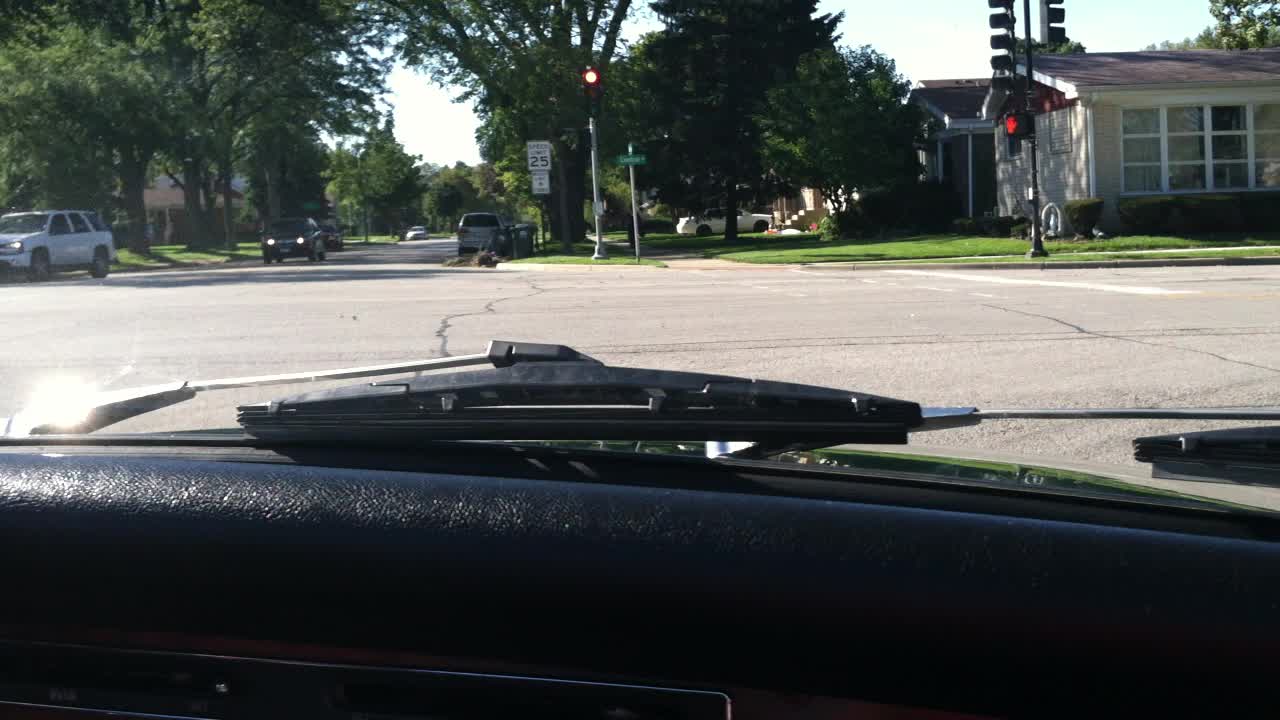This image, captured from a dash cam, depicts a spacious suburban intersection bathed in sunlight. Taken from the interior of a car with a sleek black dashboard, the scene showcases a typical sunny day with vibrant green shrubbery and meticulously maintained houses surrounding the area. Ahead, two cars can be seen in the distance, with the one in front waiting patiently at a red light. The wide street, composed of light beige-gray asphalt, is highlighted by the sun's rays streaming down onto the car's windshield wiper. Additionally, a street lamp across the road features a speed limit sign indicating a 25 miles per hour zone, further emphasizing the tranquil, residential nature of the neighborhood.